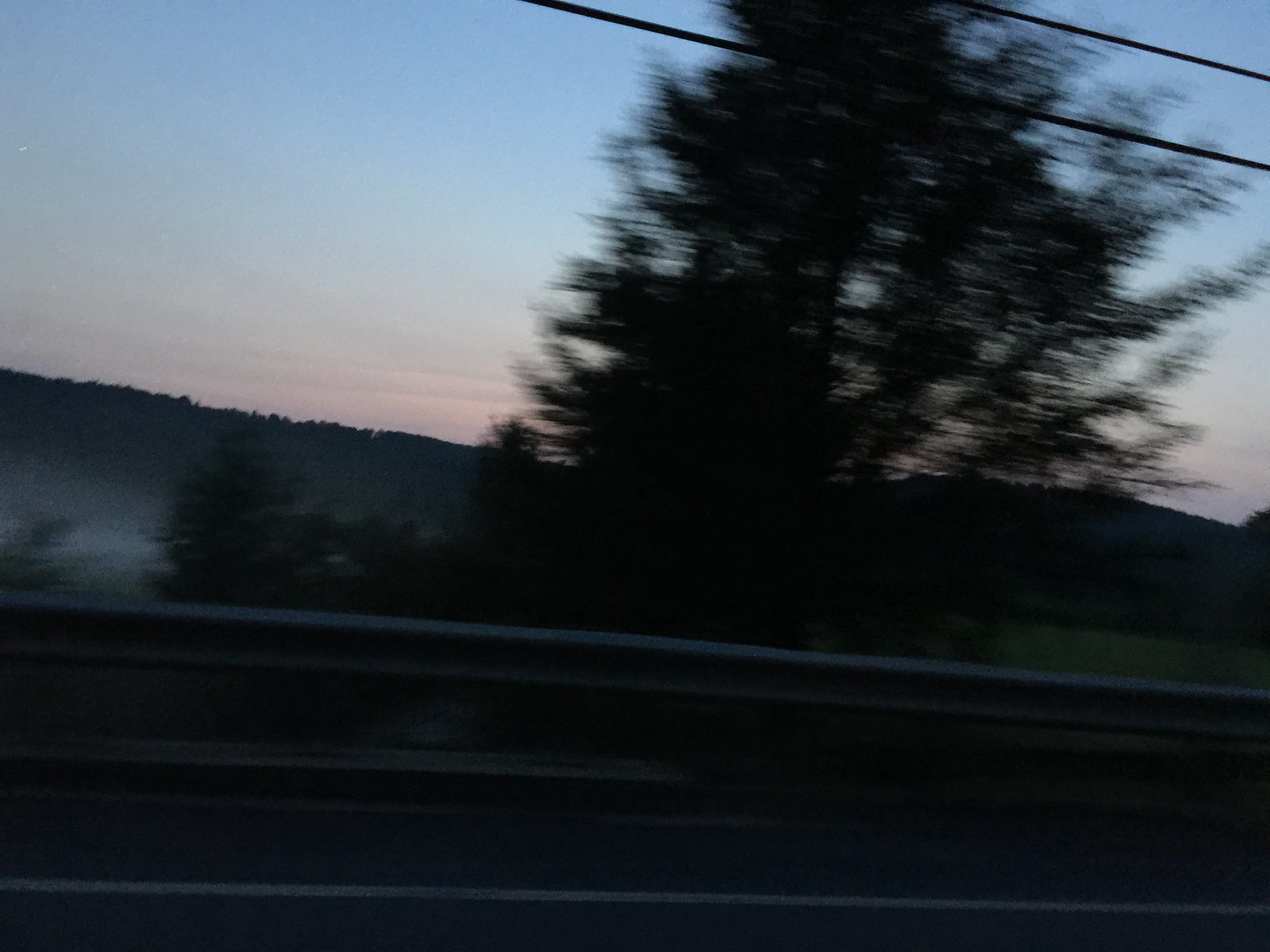A blurry photograph captures the scene from what appears to be a highway journey, with a guardrail on the roadside hinting at fast movement. Dominating the upper portion of the image is a towering evergreen tree, partially obscured by what could be a power line. The sky is a captivating blend of blue and purple, suggesting the sun is setting. Wispy clouds add a delicate texture to the dusk atmosphere. In the distant background, a dense line of trees hints at a location in or near a mountainous area, adding to the serene yet dynamic feel of the landscape.